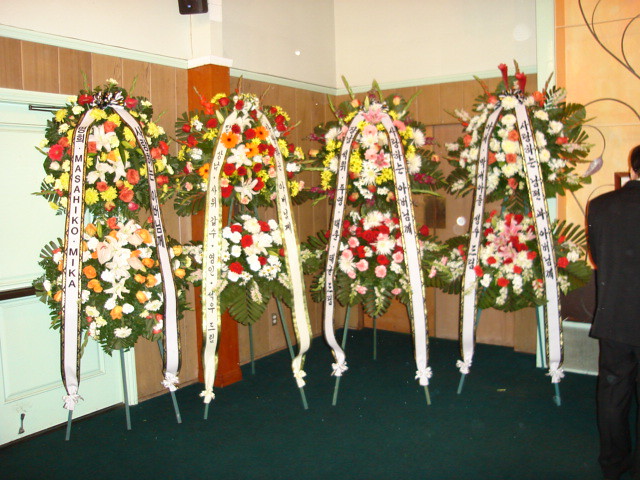This is a detailed photograph taken indoors, likely in a church-like building or conference room that could be hosting a ceremony such as a funeral. The image features four very large, ornate flower wreath arrangements standing on greenish tripods. Each arrangement consists of two stacked wreaths – one on top and one on the bottom – making for a total of eight wreaths. The floor beneath them is a dark green to black color, possibly carpeted. 

Behind the wreaths, there is wood paneling and white walls. Each wreath is adorned with a giant ribbon, which appears to have white background with gold trim. The first visible sash reads “Masahiko Mika” with Japanese-style characters next to it, while the other sashes also display similar characters. The flowers themselves are colorful, featuring shades of red, orange, yellow, pink, and white. 

On the far right of the image, there is a partially visible man in a black suit. He is seen from the back, with short dark hair, standing next to a banner, suggesting a formal atmosphere. This detailed and vibrant display suggests a significant commemorative occasion.